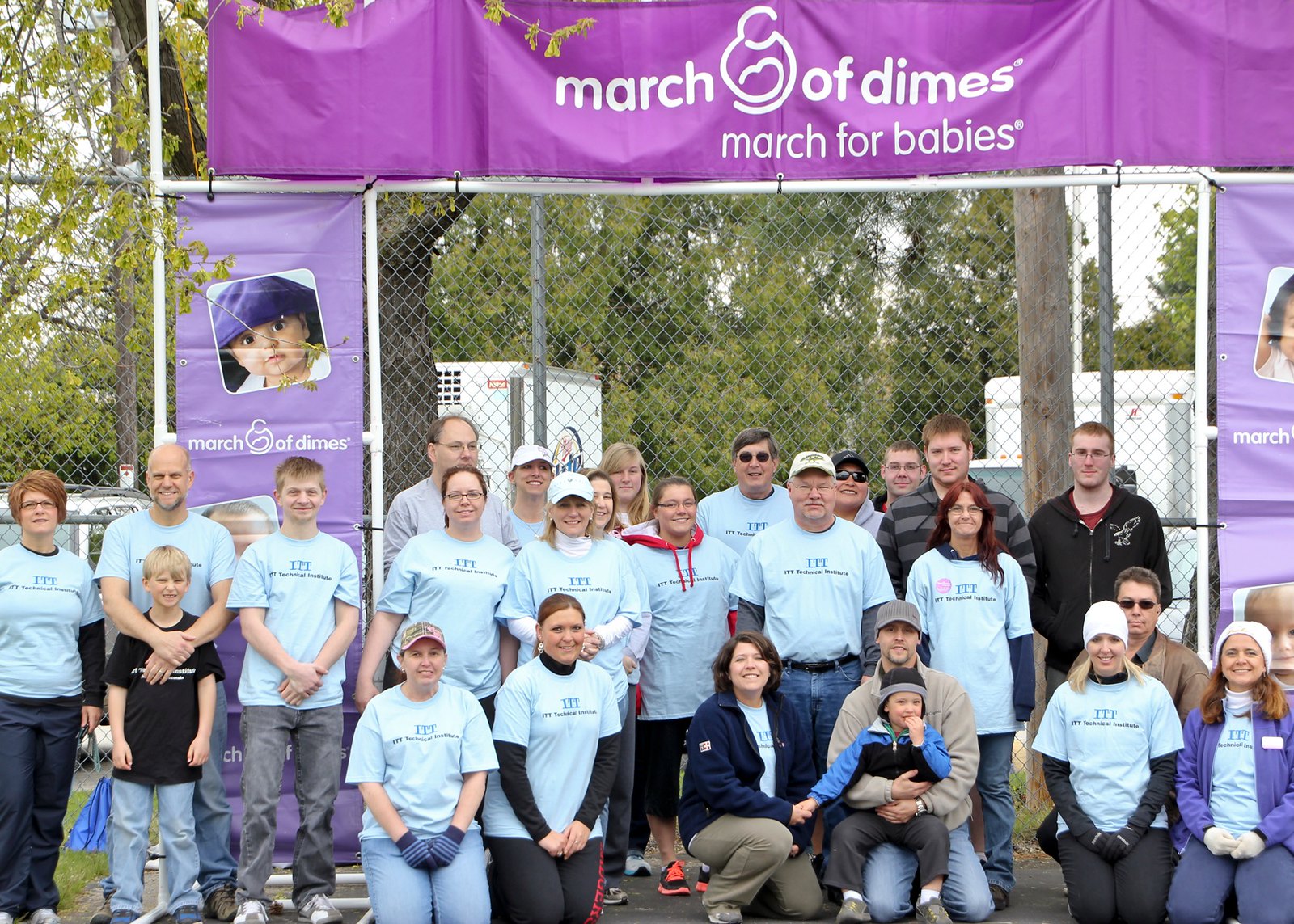In this vibrant group photo, a lively gathering of approximately 25 individuals—men, women, and children—stands prominently in front of a chain-link fence and under a prominent purple banner that reads "March of Dimes: March for Babies" in white text, complete with an image of a mother and child. The participants, most of whom are dressed in light blue T-shirts emblazoned with “ITT Technical Institute” in black text, are organized into three rows: a front row of people kneeling, a middle row of people standing, and a back row also of standing individuals. 

Interspersed among the volunteers are a few distinguished figures: a man without a T-shirt, clad in a coat, holding a young boy on his lap, while next to them, a woman kneels, wearing a blue jacket and holding another child’s hand, possibly indicating her role as the director of the event. Behind them, a chain-link fence outlines the perimeter, with white trailers visible in the distance, suggesting a parking lot background. Additional purple banners flanking the group display images of children and reinforce the cause with the "March of Dimes" name, capturing the spirited and joyful essence of these dedicated volunteers who contribute to the success of the March of Dimes initiative.